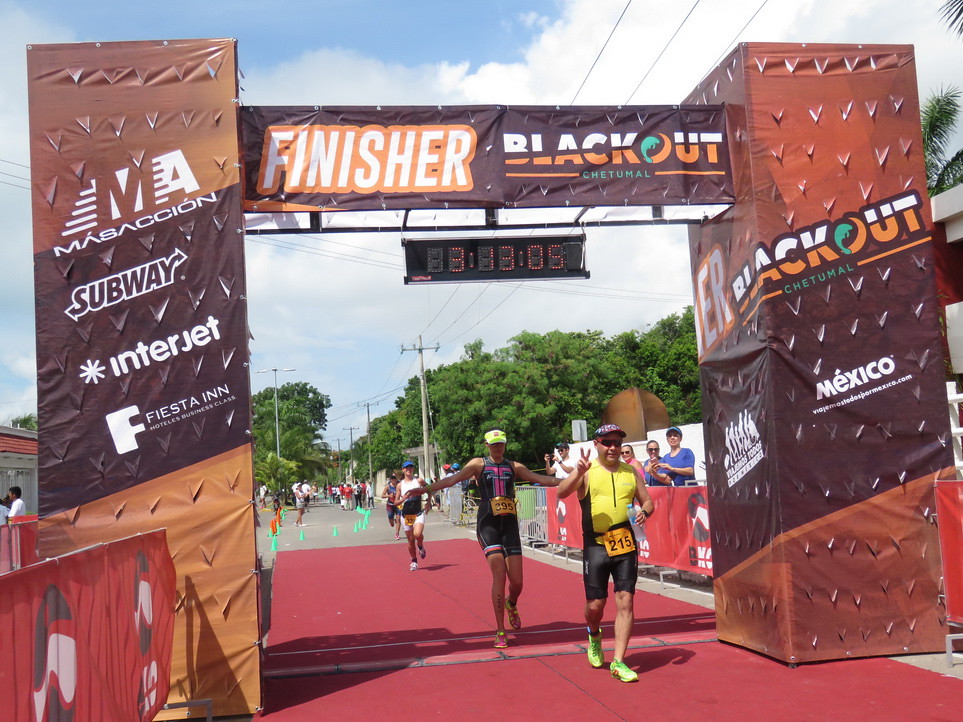The image captures the vibrant finish line of an outdoor marathon, set against a clear blue sky dotted with puffy white clouds and some patches of gray in the background. Tall green trees frame the scene in the distance, along with visible power lines. Dominating the lower portion of the image is a red carpet laid out on the street, flanked by green and orange traffic cones. Three runners are prominently featured on this red carpet: a man in a yellow and black jersey with the number 215, who has just crossed the line, followed closely by a woman in black with the number 395. Behind them, other runners are approaching. 

The finish line is defined by two vertical rectangular banners on either side, displaying the names and logos of sponsors such as Subway, Interjet, Fiesta Inn, and Blackout, Chetumal, Mexico, in alternating shades of brown. Overhead, a large banner with the words "Finisher" and "Blackout Chetumal" adorns the gateway, constructed of brown fabric over a metal frame. The gateway also features a digital time display reading 3 hours, 13 minutes, and 5 seconds. This dynamic and detailed scene captures the culmination of an intense race, highlighting both the athletes and the vibrant supporting environment.